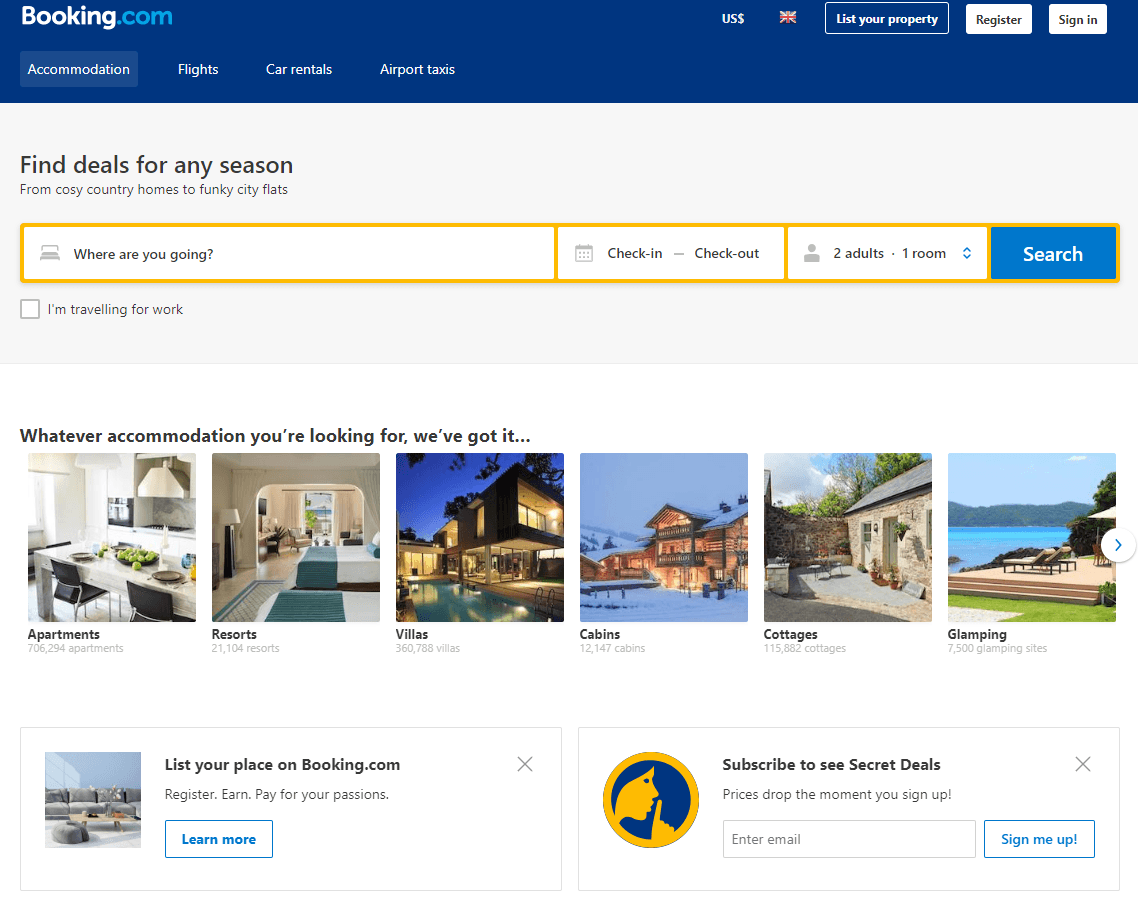Screenshot of the Booking.com Homepage:

At the top of the screenshot, a dark blue banner prominently displays the Booking.com logo on the top left, and options for "US Dollars," a UK flag icon, "Mr. Property," "Register," and "Sign in" on the top right. Below the banner, a navigation menu includes tabs for "Accommodation" (which is selected), "Flights," "Car Rentals," and "Airport Taxis."

A bold headline invites users to "Find deals for any season, from cozy country homes to funky city flats." Below this, search fields prompt, "Where are you going?" with options to enter check-in and check-out dates, and a selection for "Two adults, one room." A "Search" button follows, alongside an unchecked checkbox labeled "I'm traveling for work."

The main content area showcases a variety of accommodation types with accompanying photographs:
1. **Apartments**: An image of a modern kitchen with a marble dining area and black chairs, indicating there are 706,294 apartments available.
2. **Resorts**: A luxurious bedroom with two large white beds and a window view that appears to feature the ocean, indicating 21,104 resorts available.
3. **Villas**: A striking nighttime photograph of a luxurious home with both indoor and outdoor lights illuminated, and a lap pool in the foreground, indicating 360,788 villas available.
4. **Cabins**: A cozy ski lodge surrounded by snow-covered grounds and mountains, indicating 12,147 cabins available.
5. **Cottages**: A charming gray stone cottage, indicating 115,882 cottages available.
6. **Glamping**: An inviting deck with two lounge chairs overlooking a turquoise ocean and a tree-covered hillside in the background, indicating 7,500 glamping sites available.

The bottom left of the screen encourages property owners to "List your place on Booking.com," with options to register, earn, and pay for passions, and a link to learn more. Additionally, there is a subscription invitation: "Subscribe to see secret deals. Prices drop the moment you sign up." with fields to enter an email and a "Sign me up" button.